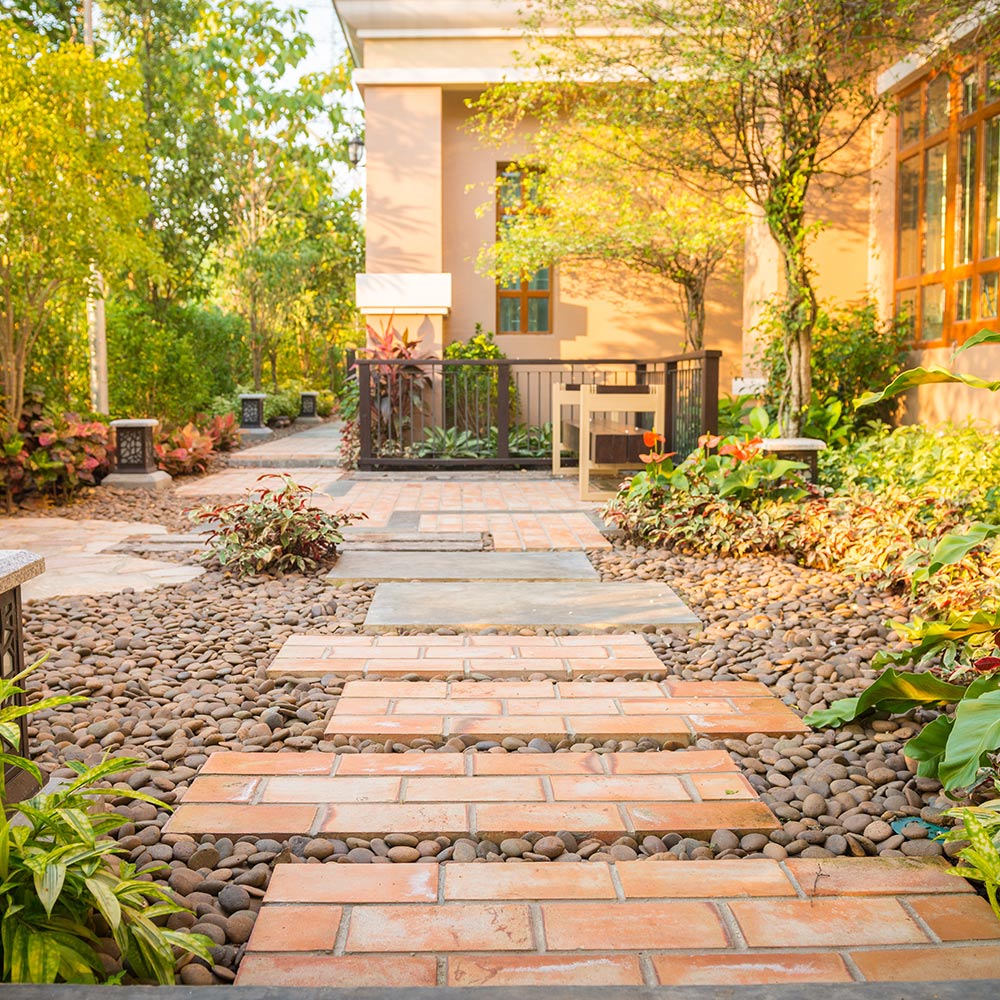This is a detailed photograph capturing a picturesque walkway of a home, possibly done in a Spanish-style with beige stucco exteriors, showcasing a blend of peach and golden-orange hues. The image predominately features a path made of light red bricks, arranged in an offset pattern, leading from the foreground to the background. These brick steps are interspersed with smooth, multicolored Mexican river rocks in shades of brown and gray, which cover the surrounding yard area.

The landscape includes an abundance of greenery—desert plants that thrive with minimal water—alongside bushes and numerous trees lining both the walkway and the side of the house, providing a lush canopy. In the backyard, there's a fence, a bench, and strategically placed pylons that appear to function as commercial-sized lights, subtly illuminating the area. Notably, there is minimal grass, indicating a low-maintenance landscape design. The photograph is framed to show just a portion of the home, including large picture windows that likely offer a scenic view of this tranquil and thoughtfully curated outdoor space.